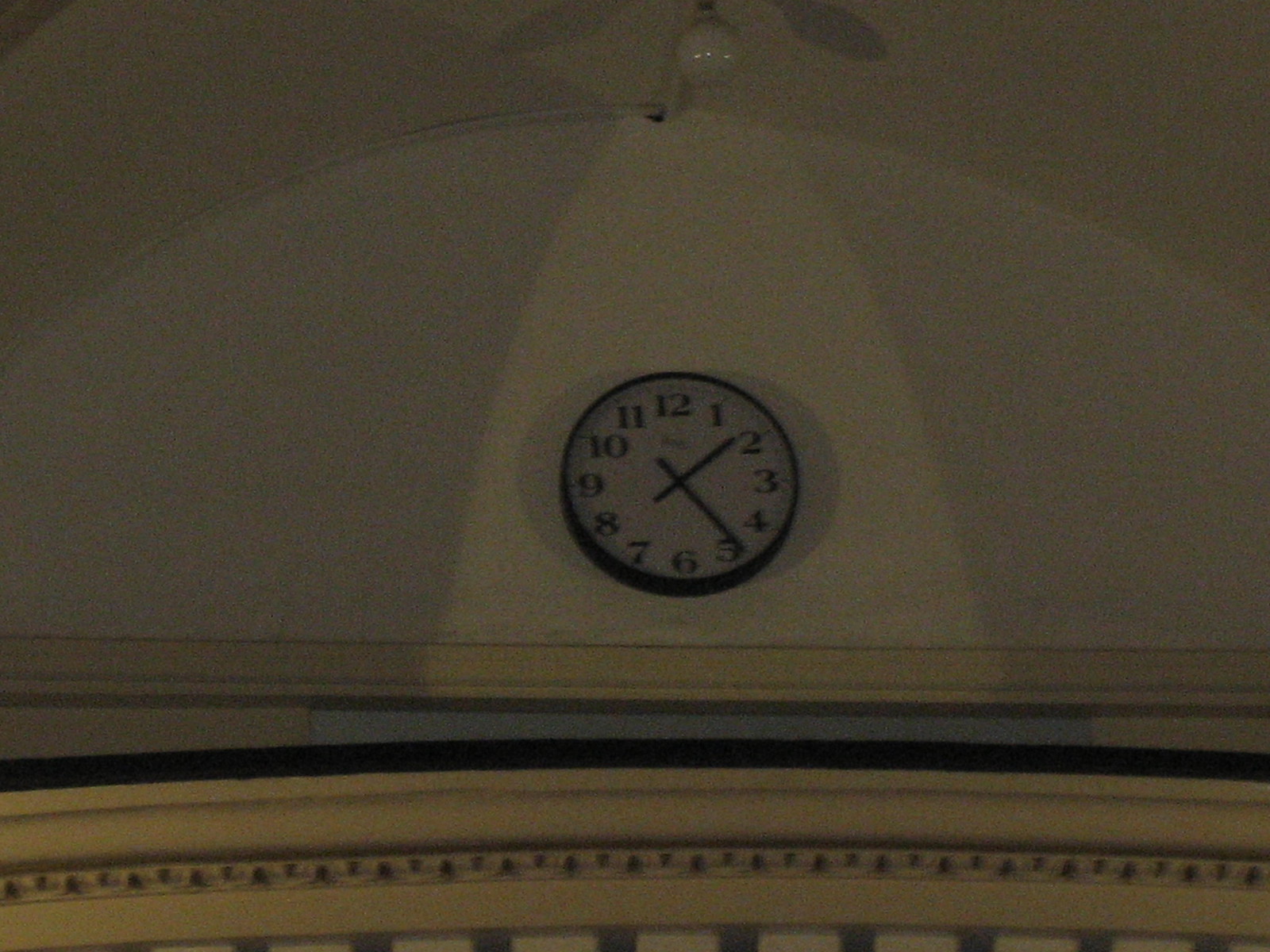The image features a wall clock prominently displayed against a distinctively striped background. The round clock, which has a black outer border and a white or cream face, shows the time as 1:25, with its little hand between the one and the two and the large hand on the five. The large, black numbers and hands stand out clearly against the lighter face. At the top of the clock, an unreadable word—presumably the manufacturer's name—sits just under the twelve. The wall behind the clock consists of a white area with beige trim at the bottom and an archway that transitions into a blue, possibly grayish segment with a patterned trim. Additionally, there's a light fixture visible at the very top of the image, showcasing a single bulb and the reflection of a ceiling fan. The overall photograph appears somewhat dark and low in resolution, adding to the intrigue of the image.